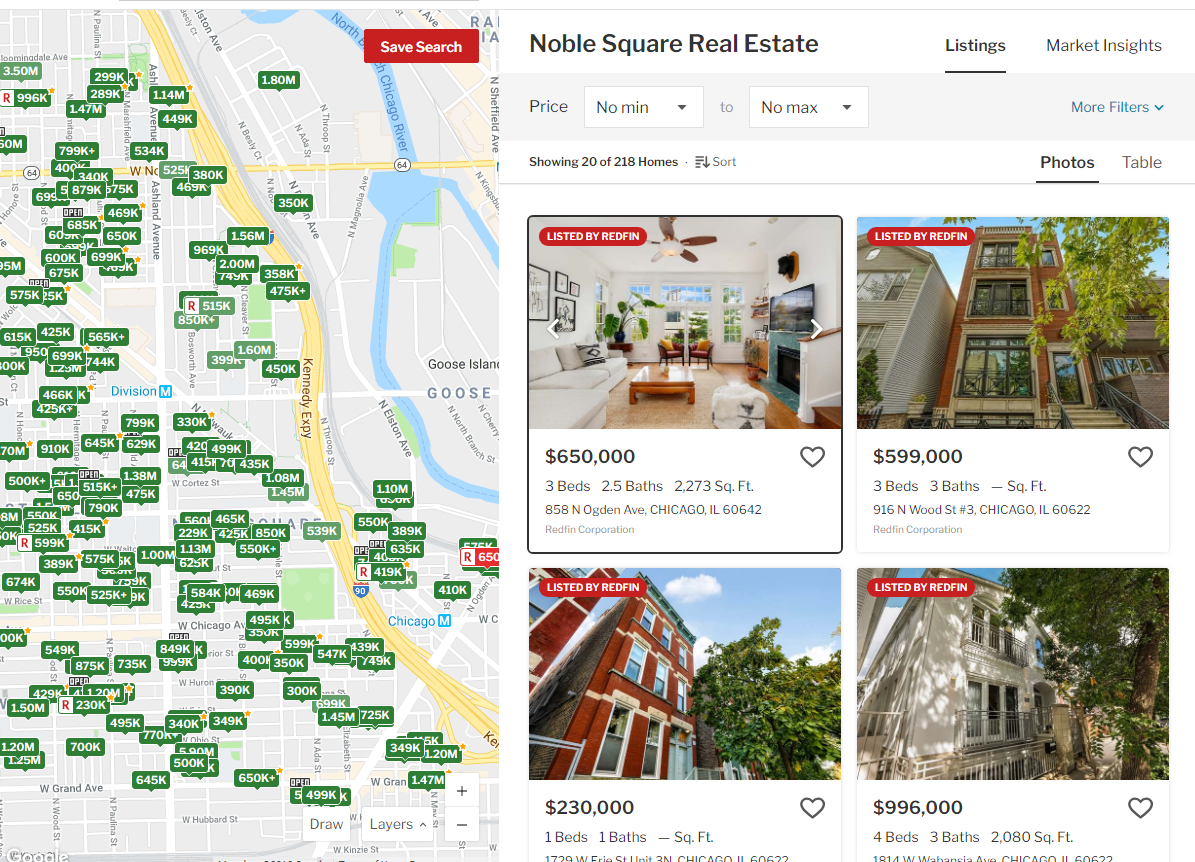The Google Maps image depicts an aerial view of expressways and streets in Chicago, specifically highlighting Ashland Avenue, Sheffield Avenue, the North Chicago River, and Goose Island. Surrounding the expressways, various properties are marked in green boxes indicating house property values, primarily ranging between $500,000 and $700,000. A notable property is denoted with a red box at the lower left, marked at $650,000, though it is partially cropped out. On the right side of the image, a real estate listing for Noble Square is visible, detailing a property priced at $650,000 with three bedrooms, two and a half bathrooms, and covering 2,273 square feet, located at 656 North Ogden Avenue, Chicago.